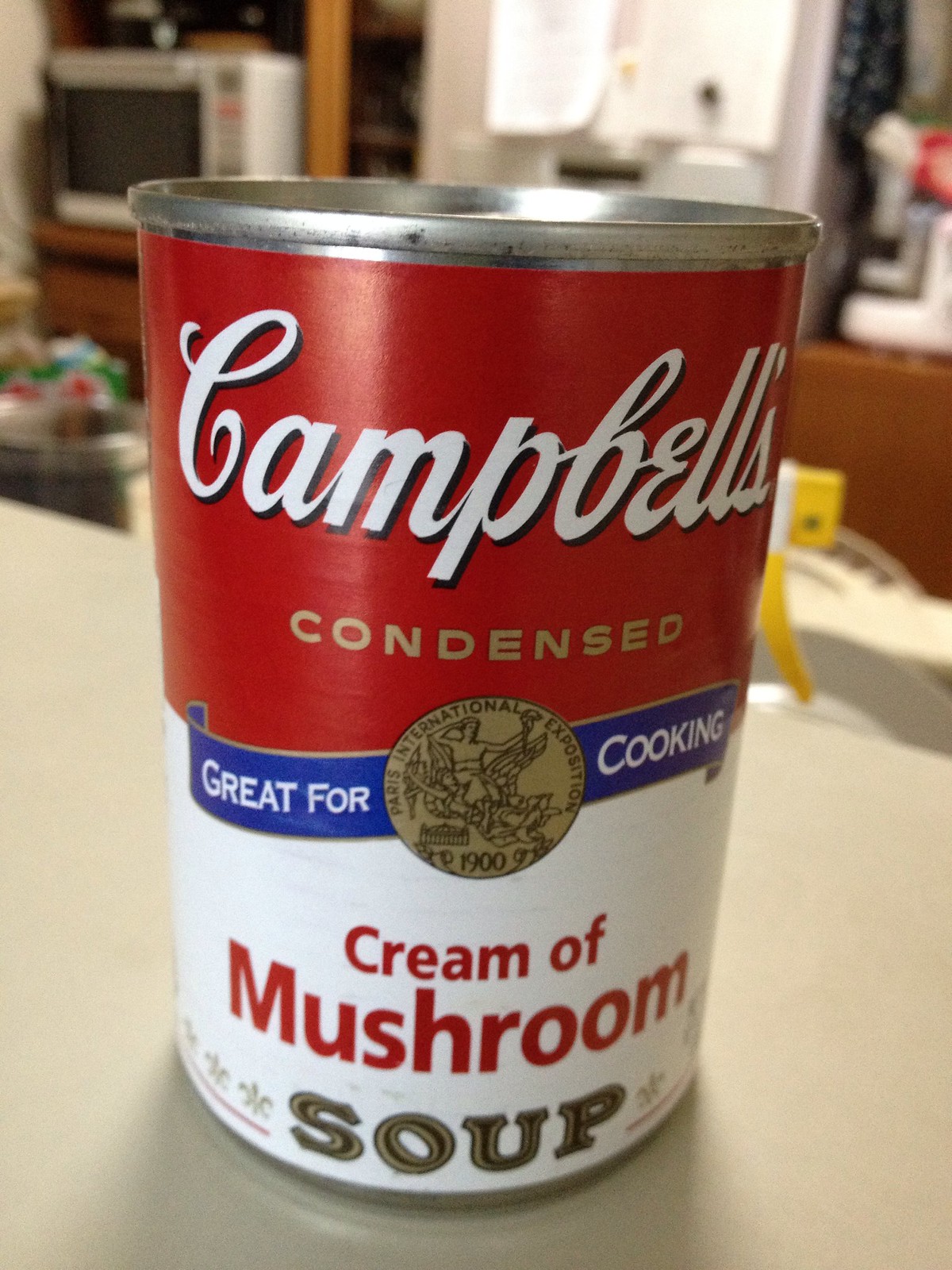A close-up of a Campbell's Condensed Cream of Mushroom Soup can dominates the foreground, sitting prominently on a white worktop. The iconic can features a red upper section with "Campbell's" in a white, handwritten-style font, and a white lower section with "Cream of Mushroom" in bold red letters and "Soup" in gold and black. A blue band across the center proclaims "Great for Cooking" in white font, alongside a gold commemorative coin from the 1900 Paris International Exposition. The can's stainless steel edges gleam at the top and bottom. In the blurred background, a typical kitchen scene unfolds with brown wooden cabinets, a microwave oven, and various indistinguishable kitchen items, offering a cozy domestic backdrop to the classic soup can.